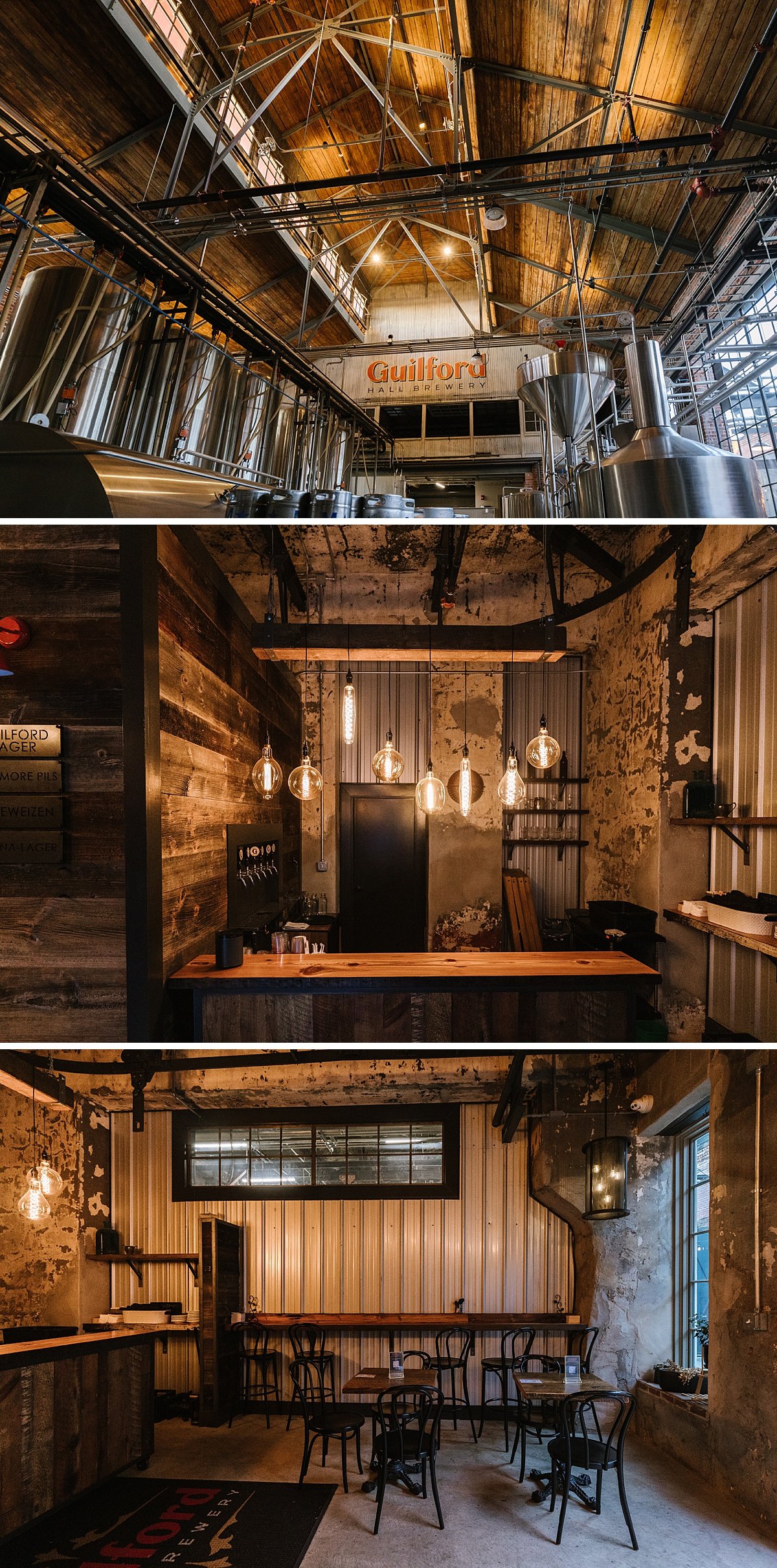The image is a stack of three photographs showcasing different interior views of Guilford Hall Brewery, emphasizing a rustic industrial farmhouse aesthetic. The top photograph captures the brewery's manufacturing area, featuring large stainless steel brewing containers with an upward view of the wooden, A-shaped ceiling supported by metal struts. A white sign with orange lettering reads "Guilford," with "brewery" discernible in black underneath. The scene is illuminated by old-fashioned lamps hanging from the rafters. The middle photograph presents a cozy tasting bar adorned with a wood top and wood paneling on the walls, illuminated by different sized lights with Edison bulbs. Exposed metal elements near the ceiling add to the industrial vibe. The bottom photograph offers a glimpse into a seating area designed for dining, with small wooden tables paired with black metal chairs and a wooden countertop bar backed by metal bar stools. This comprehensive trio of images effectively showcases the diverse spaces within Guilford Hall Brewery.